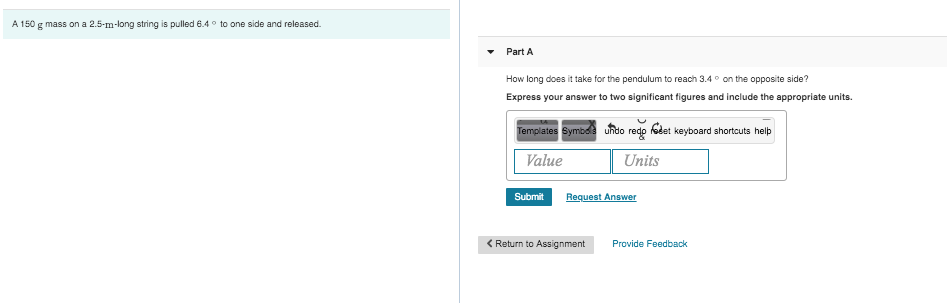A 150-gram mass is attached to a 2.5-meter-long string and is pulled 6.4 meters to one side. Upon release, the pendulum swings across to the opposite side. How long does it take for the pendulum to reach a point 3.4 meters on the opposite side? Please express your answer to two significant figures and include the appropriate units. 

(Blue box around "value" and "units.")